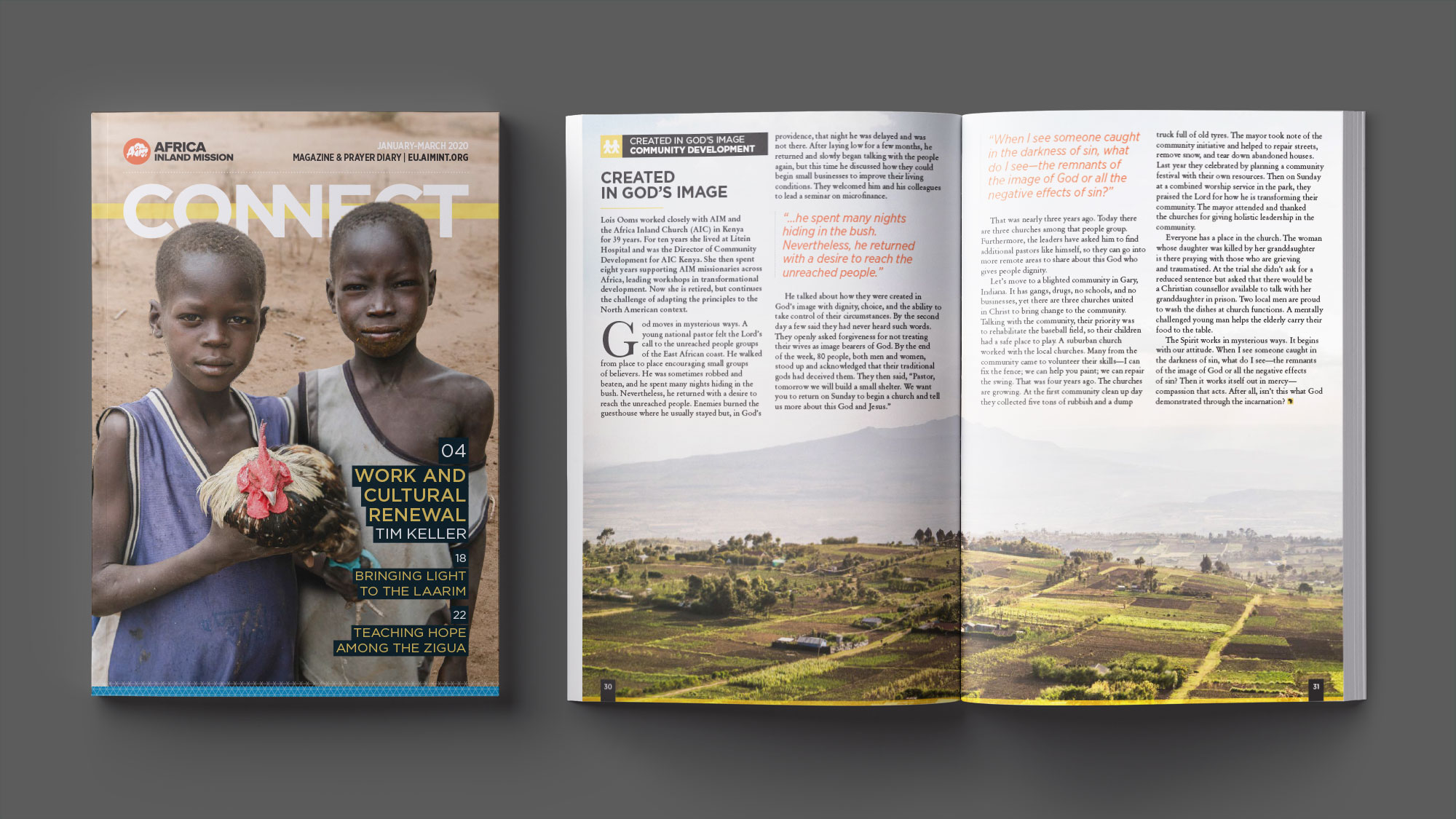The image features a magazine layout against a gray background. On the left side, the front cover of the magazine is prominently displayed. The title "CONNECT" is written in bold, white, capital letters at the top. Positioned in the upper left corner in smaller, black font is the name "AFRICA INLAND MISSION." Dominating the cover is a close-up photograph of two young African boys with very dark skin and extremely short haircuts, almost like buzz cuts. The boys have neutral expressions and are not smiling at the camera. The boy on the left is dressed in a blue tank top, while the boy on the right wears a light gray tank top that hangs off one of his shoulders. Overlaid on the image, just above the boy in the gray tank top, are the titles of some articles featured in the magazine, including "WORK AND CULTURAL RENEW" by Tim Keller.

On the right side of the image, two interior pages of the magazine are displayed. At the bottom of these pages is a panoramic photograph, likely an aerial view, depicting expansive farmland with blue mountains visible in the far distance. Although the main body text above the photo is too small to read, the headline "CREATED IN GOD'S IMAGE" stands out on the upper left side of the right-hand page. The gray background around the magazine cover and the interior pages creates the illusion that they are mounted on a gray wall.